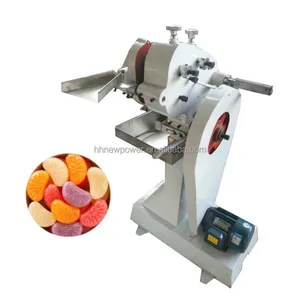The image depicts a white, metal machine reminiscent of a scientific instrument, potentially specialized for food production, such as a candy-making apparatus. This machine boasts a white base and a stainless steel chute at the top, designed for funneling materials into it. A noticeable silver handle, likely operated manually, suggests a mixing process inside the device. At the bottom, there is a small pan and a blue digital scale on the right side, implying it weighs the processed product before it's dispensed. To the left of the machine, there's a small tray filled with colorful, jelly bean-like candies in hues of orange, white, purple, and pink, suggesting this machine might be used to manufacture similar confectioneries.